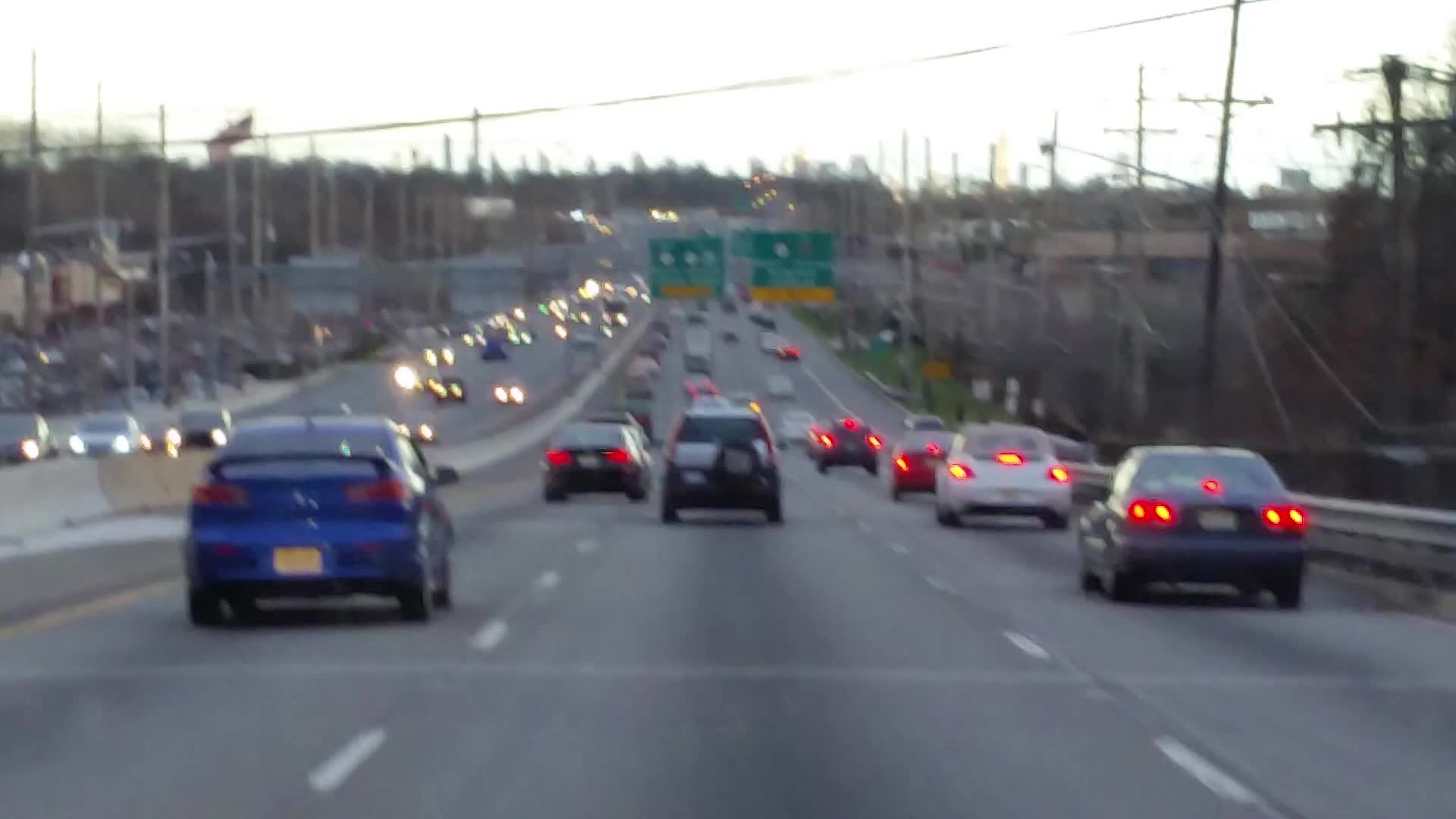This image captures a scene of a bustling freeway through the windshield of a moving vehicle in the center lane of a three-lane roadway, with three lanes visible in each direction. The photograph is slightly blurry, accentuating the motion. Ahead, a mix of cars, including an SUV, populate the lanes, while on the opposite side, oncoming traffic is seen. The freeway is lined with numerous power poles, and the surroundings are dotted with trees and buildings. To the left, a flag is faintly visible. In the distance, two large green freeway signs loom overhead, each bearing an unreadable white text and a distinguishable yellow strip at the bottom indicating "exit only" lanes. The vehicles in the rightmost lane have their brake lights illuminated, hinting at a possible slowdown or congestion in that lane.